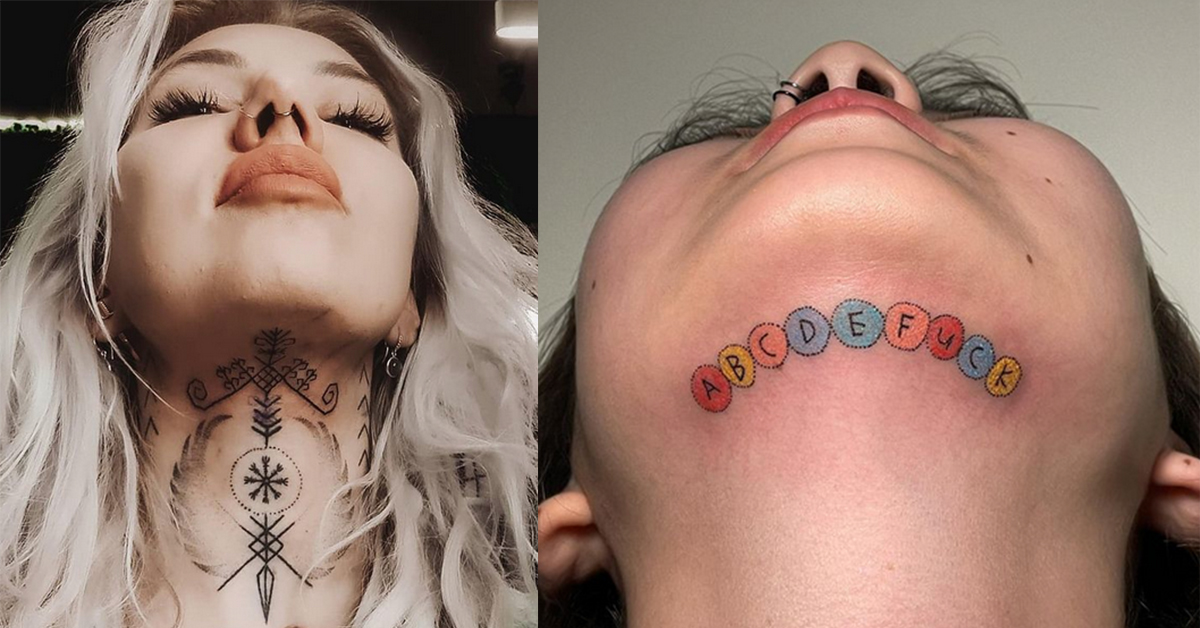This is a horizontally aligned photographic image of two similar-looking Caucasian women with distinct neck tattoos. The first woman on the left has long, almost white blonde hair cascading past her neck, thick black eyebrows, and eyelashes. She has a nose ring on the left nostril and another in the middle. Her lips are either red or pink, slightly frowning. Her head is tilted upwards, eyes closed, prominently displaying a black and white tattoo on the front of her neck. The intricate tattoo features an emblem resembling an Indian design with a snowflake-like center, surrounded by a circle, complemented by diagonal lines, vertical chevrons, and feather-like notches.

To the right is a woman with dark brown or black hair styled differently, leaning her head back to reveal a colorful neck tattoo. She also has nose rings, two on one nostril. Her lips are painted pink. The tattoo on her neck spells "A B C D E F U C K" in black letters, each encased in its own colored circle, showcasing a vibrant palette of red, yellow, pink, blue, green, and orange. Both images are similar in size and coloration, capturing the unique and striking details of each woman's tattoos and facial features.